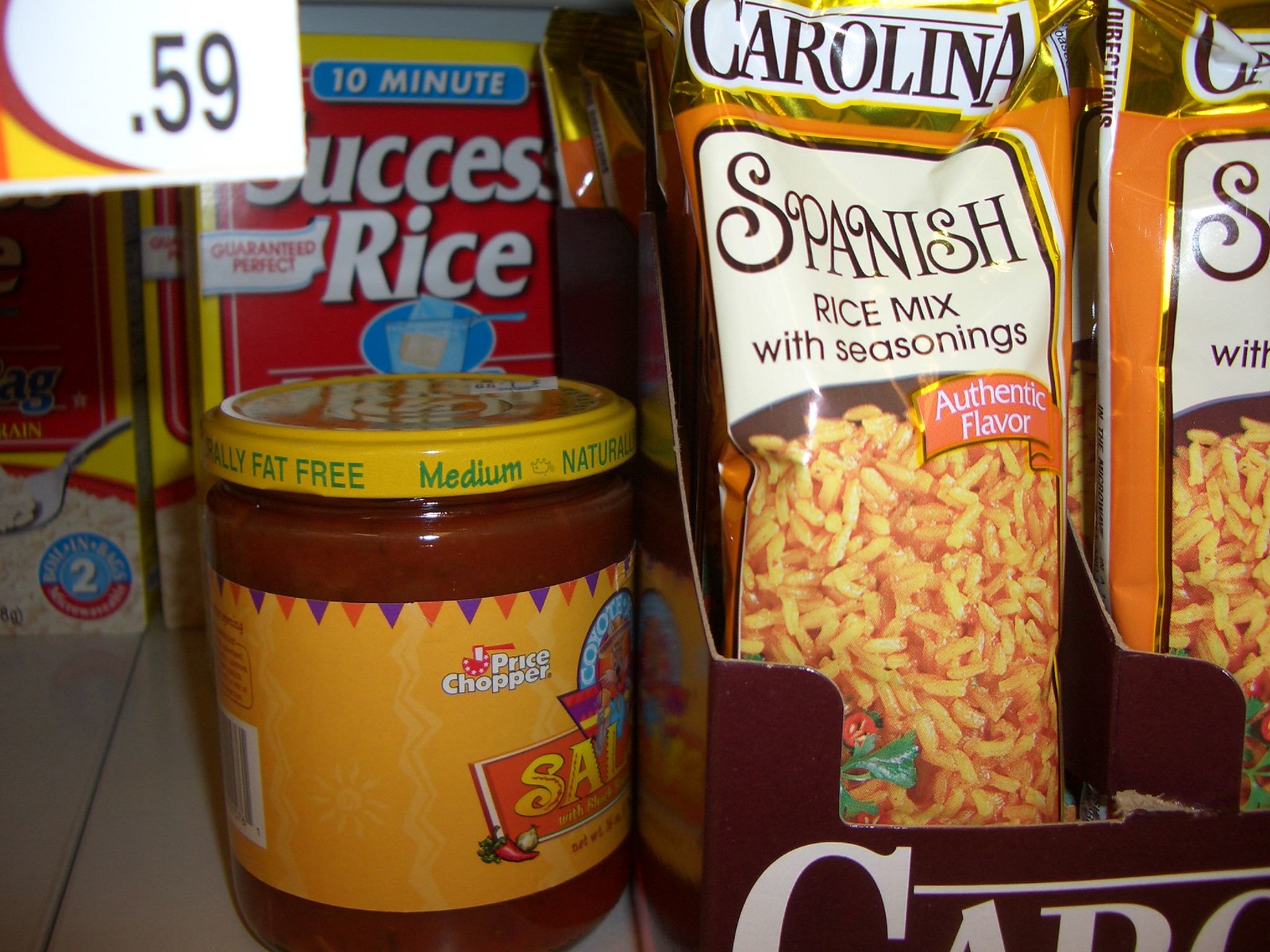The image depicts a grocery store shelf filled with an array of Spanish products. Dominating the right half of the photo is a brown cardboard display box containing several packages of "Carolina Spanish Rice Mix," which are identifiable by their orange and gold detailing, white and brown lettering, and an image of cooked rice. The box itself has white lettering that spells out "Carolina" along the bottom edge. Adjacent to the rice mix, in the center and towards the left, is a clear glass jar of salsa, likely from the brand Price Chopper. The jar features a yellow lid and band, with the phrases "totally fat-free," "medium," and "natural" prominently displayed in green, along with small flags in purple and red that add a decorative touch. The label on the jar is partially obscured but spells out "S-A-L," with an image of a red pepper indicating its spicy contents. Above this jar, to the upper left corner of the image, hangs a price sticker showing "59 cents" with a touch of yellow and a red swoop. Further to the left, another package of "10-minute Success Rice" is visible, featuring a yellow background with red and white lettering and an image of rice on a spoon. The lighting appears to be from fluorescent tubes, casting a typical indoor store ambiance.